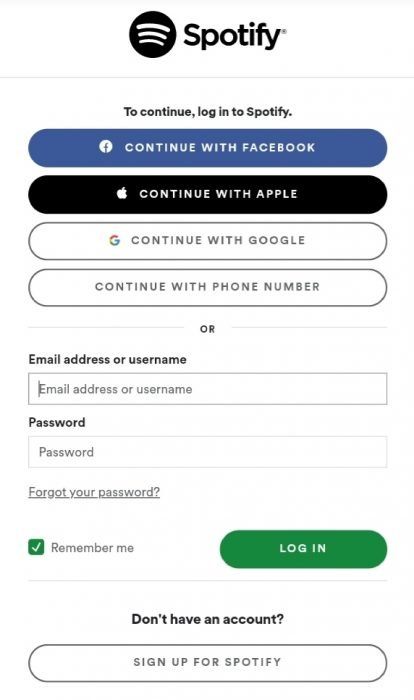The image presents a user interface for logging into Spotify within a vertical rectangular box. At the top, there is a navy circle featuring the Wi-Fi symbol. Directly beneath this, "Spotify" is written in navy blue font, with a small trademark symbol positioned above the 'Y'.

Below the logo, a prompt in small print instructs the user: "To continue, log in to Spotify." 

Following this, there are a series of elongated ovals for different login methods:
1. A navy blue oval with the Facebook logo and "Continue with Facebook" in white font.
2. A black oval with the Apple icon and "Continue with Apple" in white font.
3. A white oval with the Google logo and "Continue with Google" in black font.
4. A white oval labeled "Continue with phone number" in black font.

A thin line runs horizontally across the interface, with the word "or" centered within the line. Underneath, in slightly bolder print, are the words "Email address or username." Below this, there are input fields for "Email address or username" and "Password," both labels in darker font. 

Further down, there is a link that reads "Forgot your password?" followed by a green box with a white checkmark labeled "Remember me". 

At the bottom of the interface is a green oval with "Log In" written in white font. Below this button, there is a prompt asking, "Don't have an account?" followed by a space with a sign-up invitation: "Sign up for Spotify."